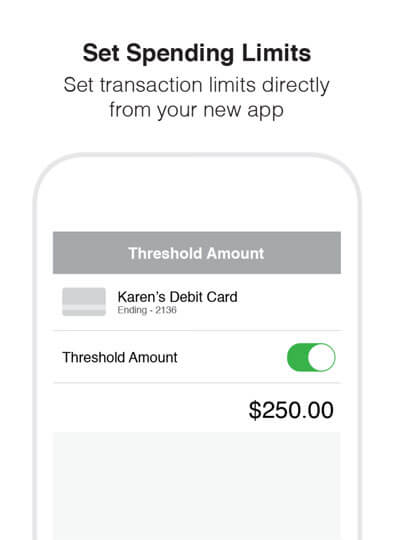Here's a cleaned-up and detailed caption for the described image:

---

The image features a mock-up of a smartphone screen against a plain white background. The smartphone is indicated by a simple gray outline, suggesting the top portion of the device. Above the mock-up, black text is prominently displayed, with the first three words, "Set Spending Limits," in bold print. Beneath this, the regular black text reads, "Set transaction limits directly from your new app."

Within the smartphone mock-up, the uppermost section includes a gray bar with white text that reads, "Threshold Amount." Below this bar, there is a small icon representing a credit card and the words "Karen's Debit Card" positioned towards the right-hand side. Alongside this, there's the word "Ending" followed by the numbers "2136."

Further down, another gray line separates the upper content from the lower section. Below this line, the text "Threshold Amount" is displayed again, accompanied by a green switch and a value set to "$250."

---

This detailed and organized caption captures all the key elements clearly present in the image mock-up.